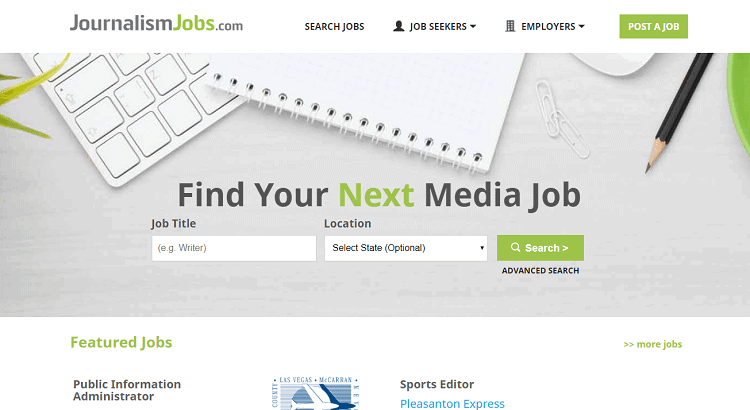The image is a screenshot of a webpage from JournalismJobs.com. At the top left corner, the text "JournalismJobs.com" is displayed, with "jobs" in green and "journalism" and "com" in gray. To the right, there are four links: "Search Jobs," "Job Seekers," and "Employers," with a green rectangle at the top right bearing white text that reads "Post a Job."

The central portion of the image is dominated by a gray rectangle featuring the edge of a keyboard, a notepad, and a black pencil in the top right corner. Prominently displayed in the middle of this section is the phrase, "Find your next media job," with "next" highlighted in green and the rest in gray. Below this, there are three user input fields labeled "Job title" (with a fill-in bar), "Location" (with a drop-down menu), and a green rectangle labeled "Search" in white text. Directly under these fields is a small text link reading "Advanced Search" in black.

At the bottom of the page, the background turns white and features a section labeled "Featured Jobs" in green text at the top. In the bottom left corner of this area, the job title "Public Information Administrator" is listed in black text. In the top right corner of this section, green text reads "More Jobs," accompanied by two right-facing arrows. Centrally located at the very bottom is a light blue icon featuring an airplane, with text reading "Las Vegas, McCarran" in light blue. Next to this icon are the text entries "Sports Editor" in black and "Pleasanton Express" in light blue.